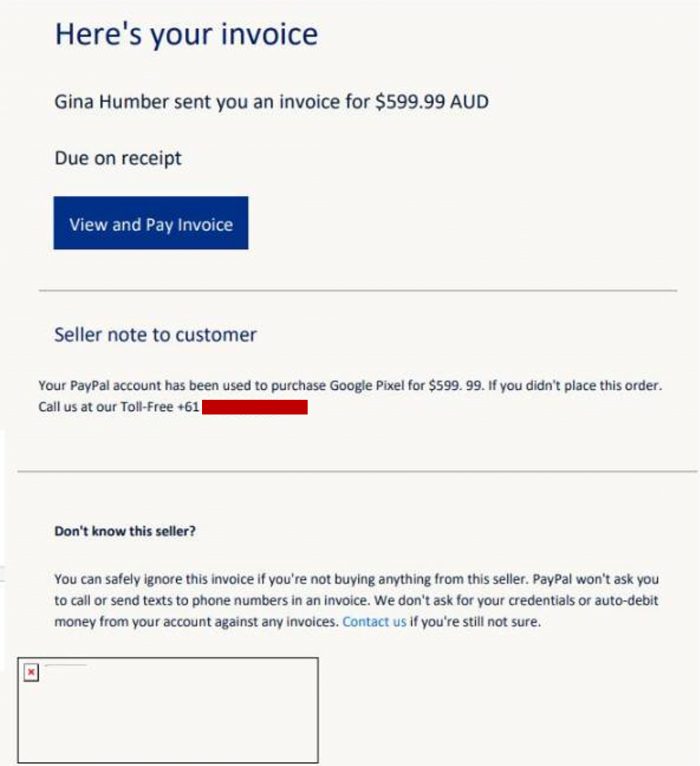This image is a cropped screenshot of an invoice box from a web page. At the top left, bold blue text announces, "Here's your invoice." Directly below it, the invoice details state, "Gina Humber sent you an invoice for $599 AUD." The next line emphasizes, "Due on receipt" in bold blue letters. Beneath this information, there is a rectangular button on the left labeled "View and Pay Invoice."

In the center of the box, it reads "Seller note to customer." Following this, a detailed note specifies: "Your PayPal account has been used to purchase Google Pixel for $599.99. If you didn't place this order, call us at our toll free." However, the actual phone number is obscured by a red box. 

Towards the bottom, a section titled "Don't know the seller" provides a cautionary notice, with a blue hyperlink stating "Contact us" embedded within the paragraph. 

In the bottom left corner of the screenshot, there's an empty box with a broken image icon, indicated by a red X in the upper left corner of the box. The entire background of the image is a muted gray, adding a somber tone to the overall layout.